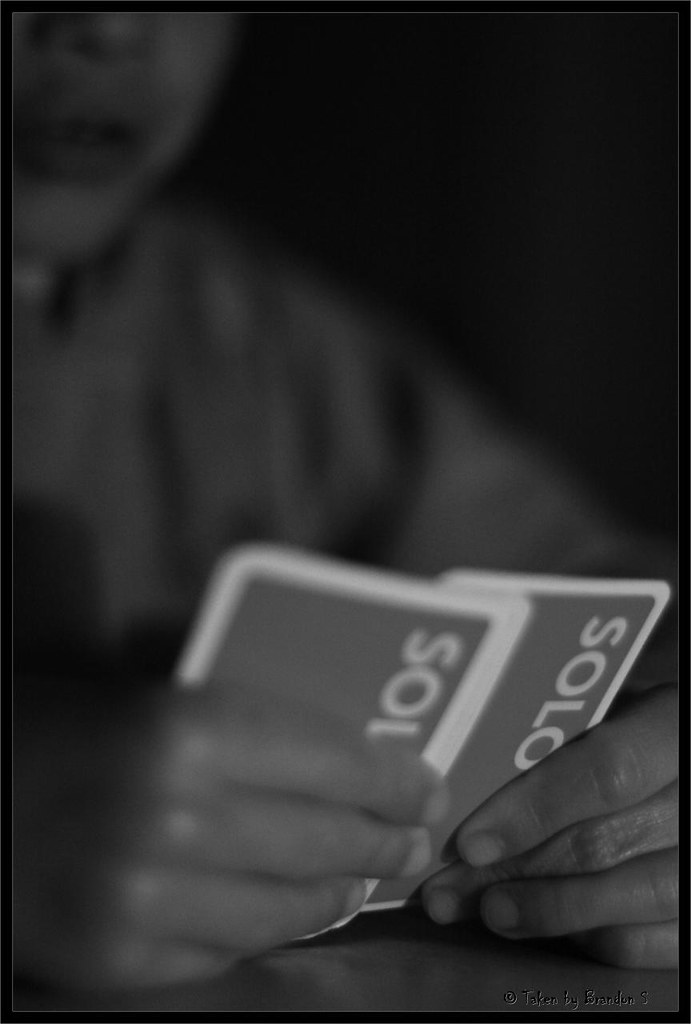A black and white photograph captures a moment steeped in mystery. The image is mostly out of focus, lending it an abstract, almost dreamlike quality. Dominating the frame is the lower half of an individual's face, with their mouth slightly ajar, hinting at a pensive or concentrated state. The person is casually clad in a t-shirt, the soft fabric barely discernible in the low light. 

In the foreground, the well-lit fingers of the person's left hand come into sharp focus. The hand is holding at least three playing cards. We see the backs of these cards, which feature a prominent white border. Two of the visible cards are marked with the word "Solo," though any additional text is obscured. The individual's gaze appears fixated on the cards they hold, lost in a private moment of contemplation or strategy.

At the very bottom of the image, a small watermark reveals the photographer's signature: a circle enclosing a 'C' for copyright, followed by the relaxed script of "taken by Brandon S." The overall darkness of the image adds to its enigmatic atmosphere, inviting viewers to ponder the unseen face and the story behind the cards.